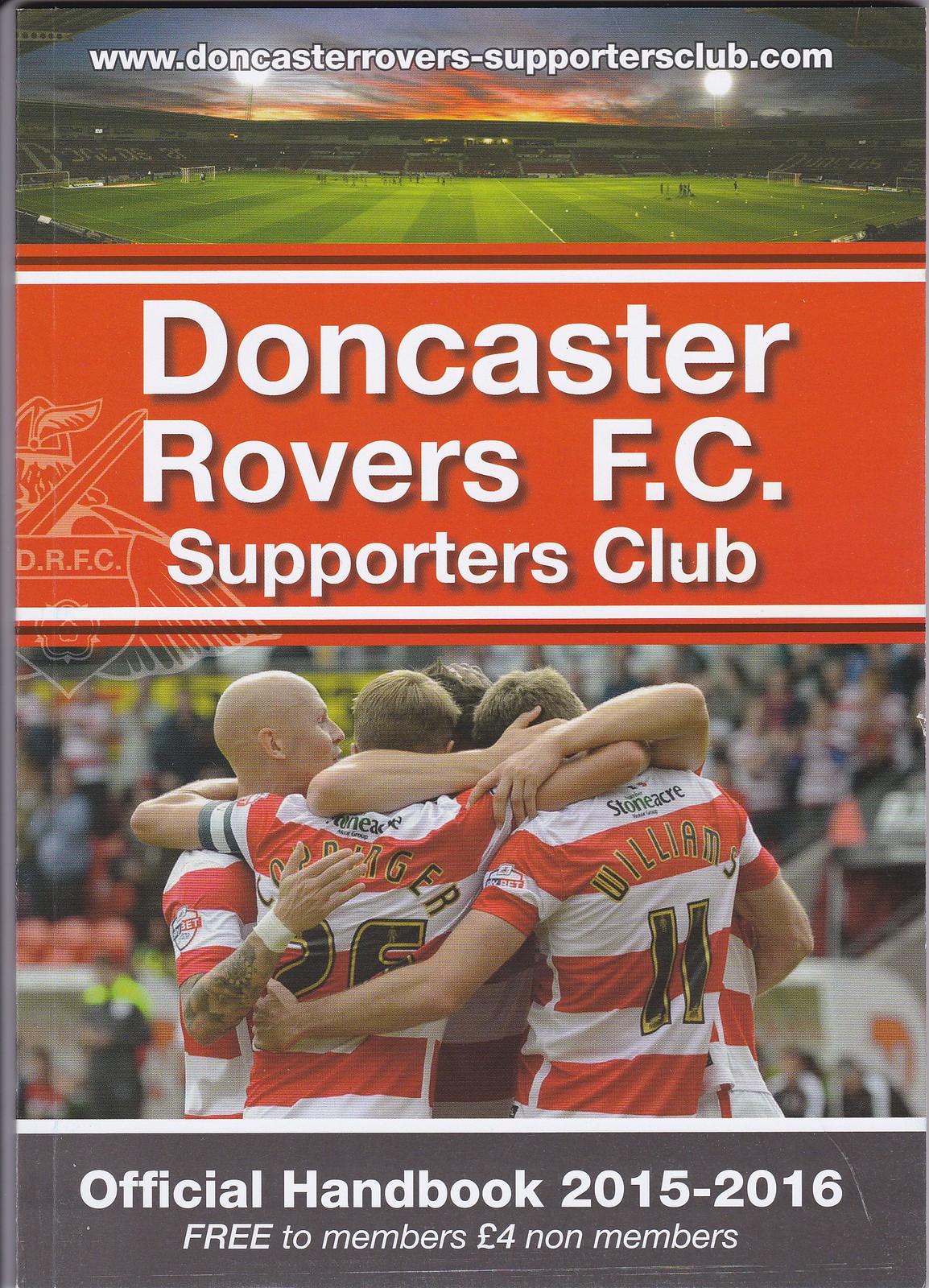This is the cover of a football program in color, showcasing a detailed layout from top to bottom. At the very top, set against a background that blends a distant soccer field meeting the sky, is the web address "www.doncasterrovers-supportersclub.com" in white letters. Just below this, a prominent red banner spans across the booklet, with the words "Doncaster Rovers FC Supporters Club" in bold white font. Moving to the bottom half of the cover, a scene captures four football players in a close embrace, all wearing white and red striped jerseys with numbers on their backs. They celebrate in front of an audience visible in the background, with spectators filling the stands. The bottom of the program features a gray border that reads "Official Handbook 2015-2016 – Free to members, Four pounds for non-members."